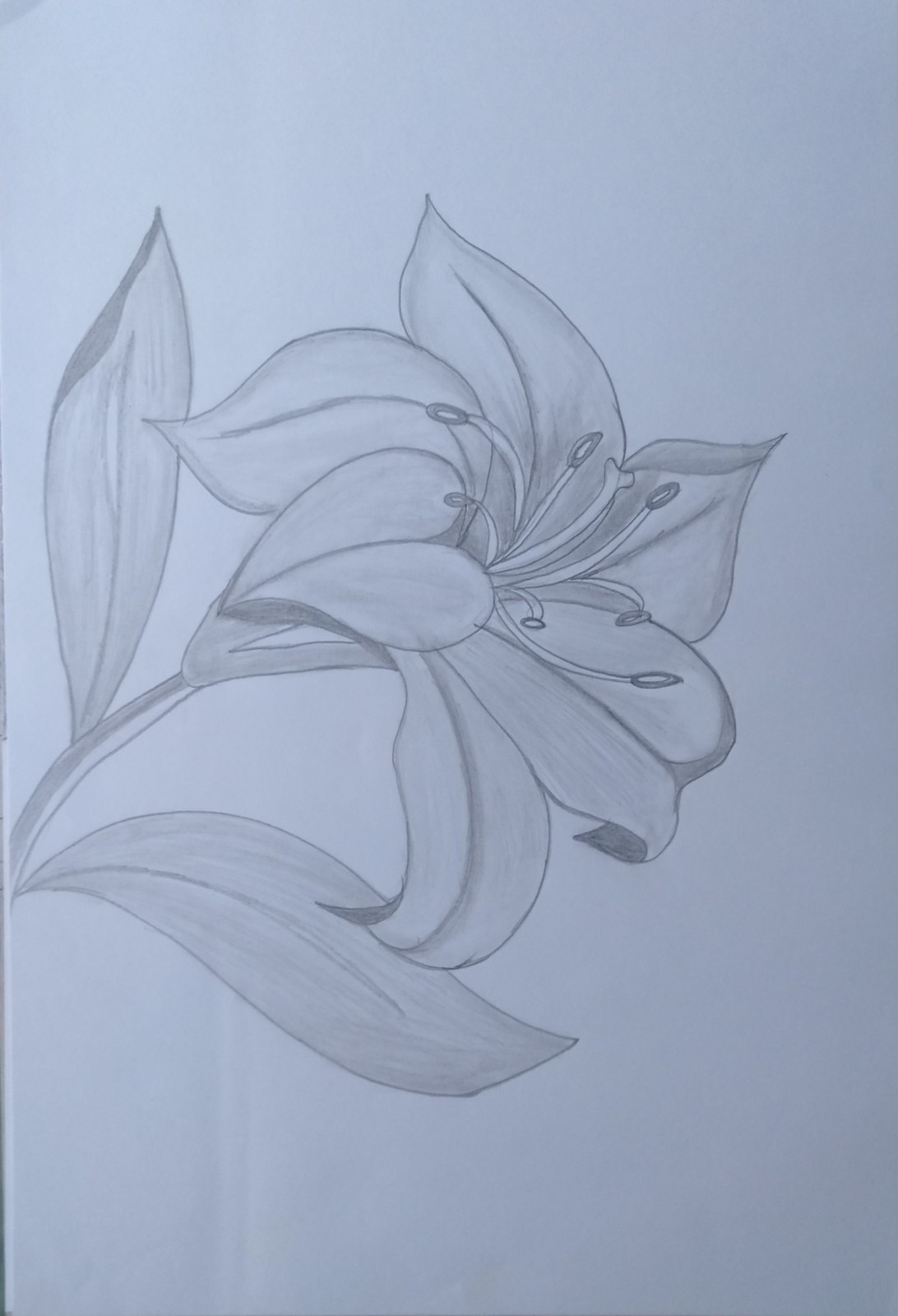This detailed pencil drawing of a beautiful flower is rendered on a light-colored piece of paper. The flower, reminiscent of a lily, features six elongated petals that unfurl gracefully. The petals exhibit a blend of smooth curves and slight pointed tips, with subtle shading giving them depth and dimension. 

Emerging from the center of the flower are seven stamens with small buds on their tips, along with one additional stamen without a bud. This creates a striking focal point. The flower is attached to a single, sturdy stem with two large, detailed leaves at the base. One of the leaves has a slight curl at the tip, accentuated by meticulous shading that brings out the intricate vein patterns.

The overall composition is oriented sideways on the paper, offering a unique perspective of the flower’s form and structure. The artwork's monochromatic pencil rendering showcases the artist's precise technique and ability to convey texture and intricacy without the use of color.